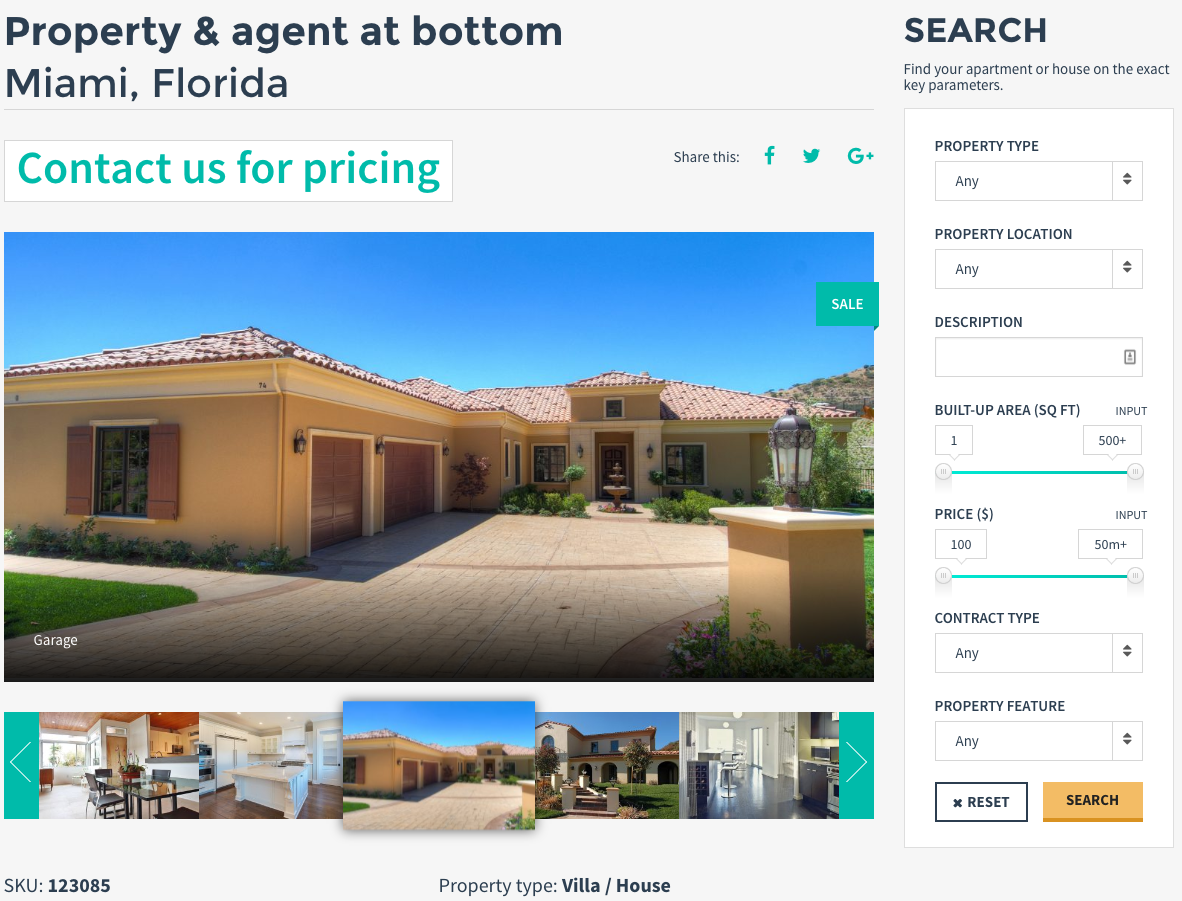Here’s a cleaned-up and detailed caption for the described image:

---

This vertical image features a flat gray background with no texture or dimensional elements. At the top left, bold black text reads "Property and Agent," with a slightly bolder subtitle, "Miami, Florida," beneath it. A thin gray line extends horizontally, separating this section from a white box with a seafoam green background, where "Contact Us for Pricing" is written.

On the right side of this section, there are options to share the property listing via Facebook, Twitter, or Google+. Below this, an outdoor image of the home is displayed, showing a clear blue sky, green grass, and distant mountains in the background. Green arrows at the bottom corners of the image allow users to browse more photos of the home’s interior and exterior.

At the bottom of the page, a SKU number is provided, along with the property type labeled as "Villa/House." In the upper right corner, a search bar is available with an option to "Find Your Apartment or House on Exact Key Parameters," allowing searches by property type, location, description, built-up area, square footage, price, contract type, and property features. Users can reset the search or initiate it by pressing the respective buttons.

---

This caption provides a comprehensive and detailed description of the image, maintaining clarity and organization.